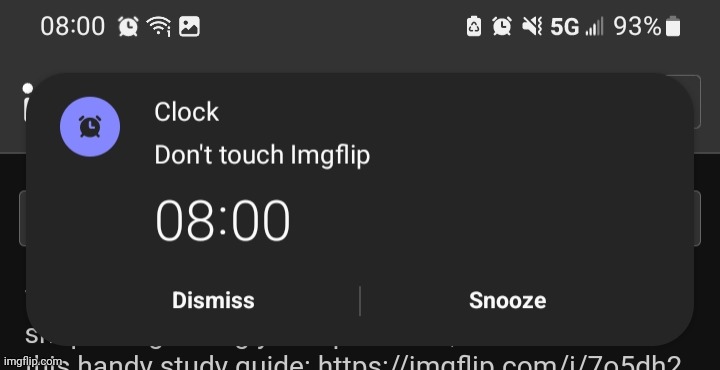This image is a screenshot taken from a cell phone with a black background. At the top, in white text, it displays the time as "08:00" alongside an alarm clock icon in white. Additionally, there is a Wi-Fi signal symbol next to an eye icon. Further along from left to right, there is a square icon with a black circle and a mountain-like shape at the bottom, followed by symbols for battery status, another alarm clock, and a volume icon with a diagonal line through it, indicating muted sound. The status bar also shows "5G" with a capital G, a cell signal indicator, and a battery percentage at "93%".

Below this, partially visible text and graphics are cut off, likely due to a dark-colored pop-up overlaying the screen. This pop-up includes a prominent, bright purple circle with cooler, blue undertones. Adjacent to the purple circle, in larger text, it says "Clock" with the C capitalized. Underneath, it reads "Don't touch" followed by "LMG flip". Further down, it indicates the time again as "08:800". At the bottom of the pop-up are two options: "Dismiss" or "Snooze".